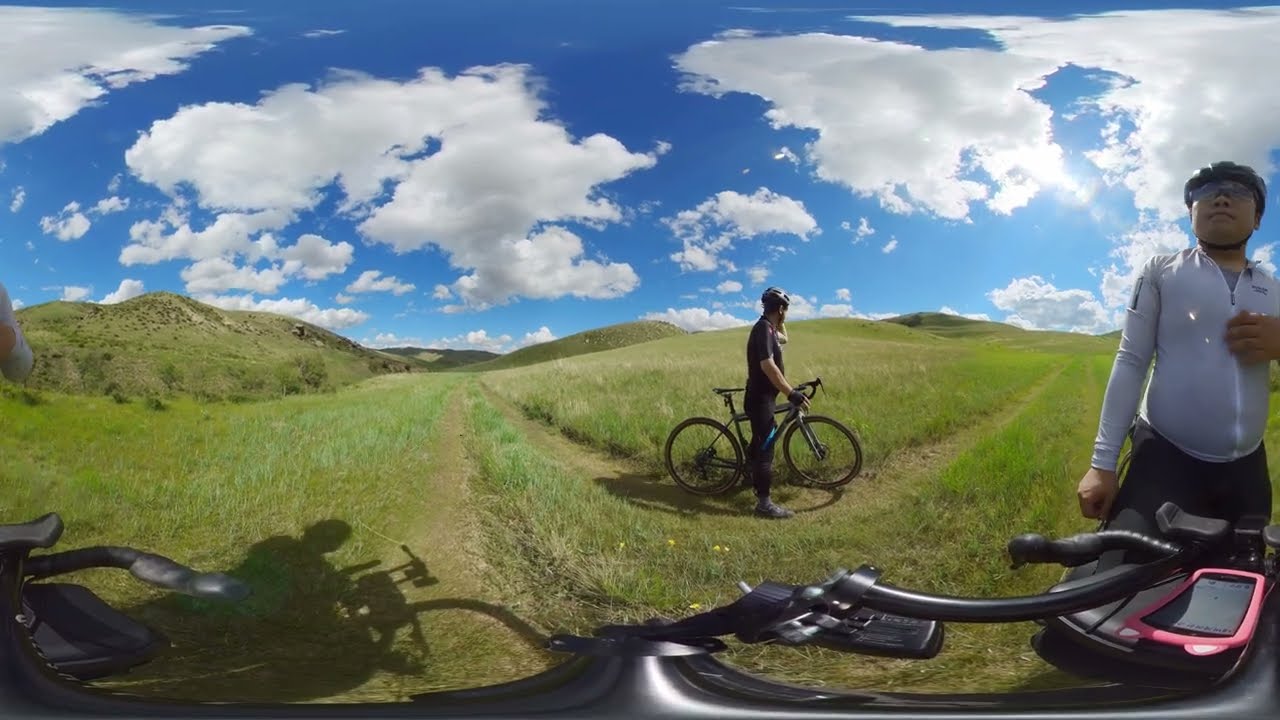The image captures a panoramic view from the helmet-mounted GoPro of a cyclist, revealing a grassy field with a trodden path cutting through it. In the foreground, handlebars can be seen, emphasizing the cyclist's perspective. Slightly right of center, a cyclist in a black short-sleeved shirt, black pants, and a black helmet is seen paused on the path, looking into the distance. On the far right, another cyclist appears. He is an Asian man wearing a white zip-up sweatshirt, black pants, glasses, and a black helmet, also seemingly paused and gazing upwards. The lush, green field is complemented by rolling grassy hills and a blue sky dotted with fluffy white clouds, indicating a sunny day perfect for biking.